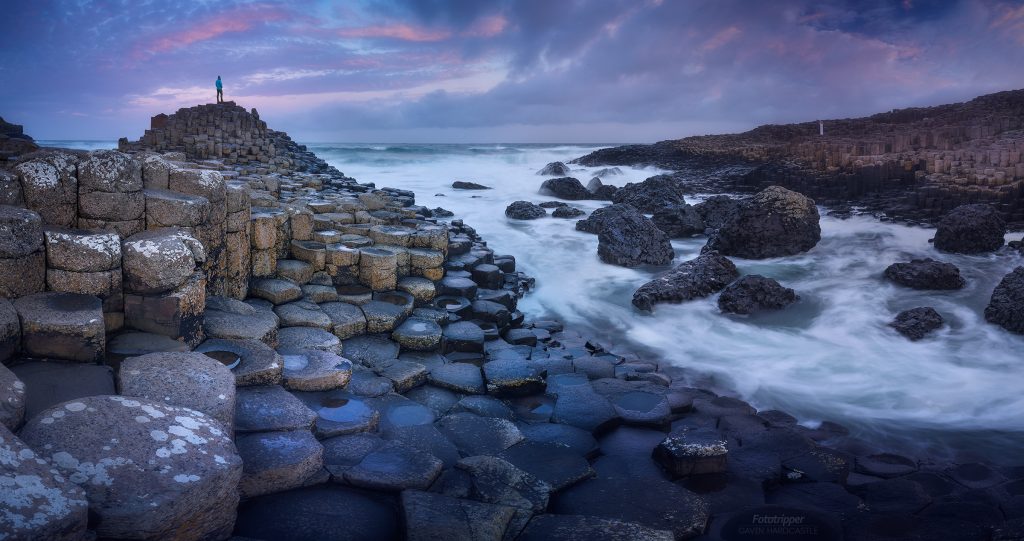The photograph captures a serene yet dramatic rocky shoreline, likely during dawn or early dusk, with subtle HDR editing enhancing its features. The image depicts an ocean scene viewed from the shoreline, where waves break over weathered rocks, creating a frothy white-capped appearance. The rocky coast extends from the right to the left, forming a slight mound on the left side, where a person stands, gazing out into the ocean. These rocks, resembling steps or columns of semi-rounded disks, have been gradually worn down over time, varying in height as they stack higher away from the water.

On the right side, there's a small inlet or cove framed by more of these distinctive rock formations. The sky above is filled with clouds, painted in a palette of purples, blues, and hints of pink and red, suggesting the sun is setting or just rising. The overall ambiance of the photograph is slightly dark, not overly bright, and evocative of a tranquil yet majestic coastal landscape, possibly reminiscent of the striking rock formations found in places like Ireland.